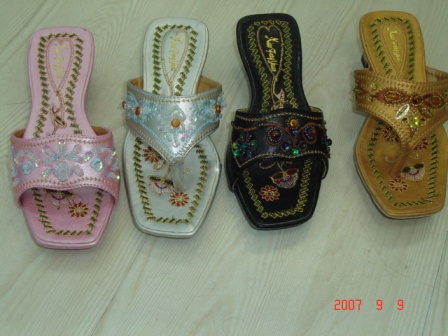This colored photograph showcases four distinct women's sandals, arranged neatly on a tan wood floor. In the lower right-hand corner, the red text "2007-99" indicates the year, month, and date. Each sandal features unique designs and embellishments, creating a vibrant display.

From left to right, the first sandal is a vivid hot pink, adorned with intricate blue, pink, and olive green floral embroidery. It features a bowling-pin-shaped design with a blend of purple, red, and pink flowers, accented by shimmering rhinestones. 

The second sandal is pearl white with a graceful V-shaped strap. It is decorated with elegant butterfly and flower embroidery around a gray strap, highlighted by iridescent jewels and gold stitching. The floral designs include shades of red, purple, and olive green.

The third sandal is black, with a simple yet striking strap. It boasts an array of floral embroidery featuring red, gray, and pink flowers, which are embellished with blue and dark blue rhinestones. The sandal also displays text in a heart shape at the back, complemented by a larger gray and red flower.

The last sandal, in a brassy golden hue, showcases a floral design with brown and yellow accents, interspersed with rhinestones. It features motifs of smiling pink and red flowers with olive green embroidery, rounding off the unique collection.

Each sandal, whether described with beads, rhinestones, or embroidery, contributes to the overall aesthetic, creating a harmonious blend of colors and designs.